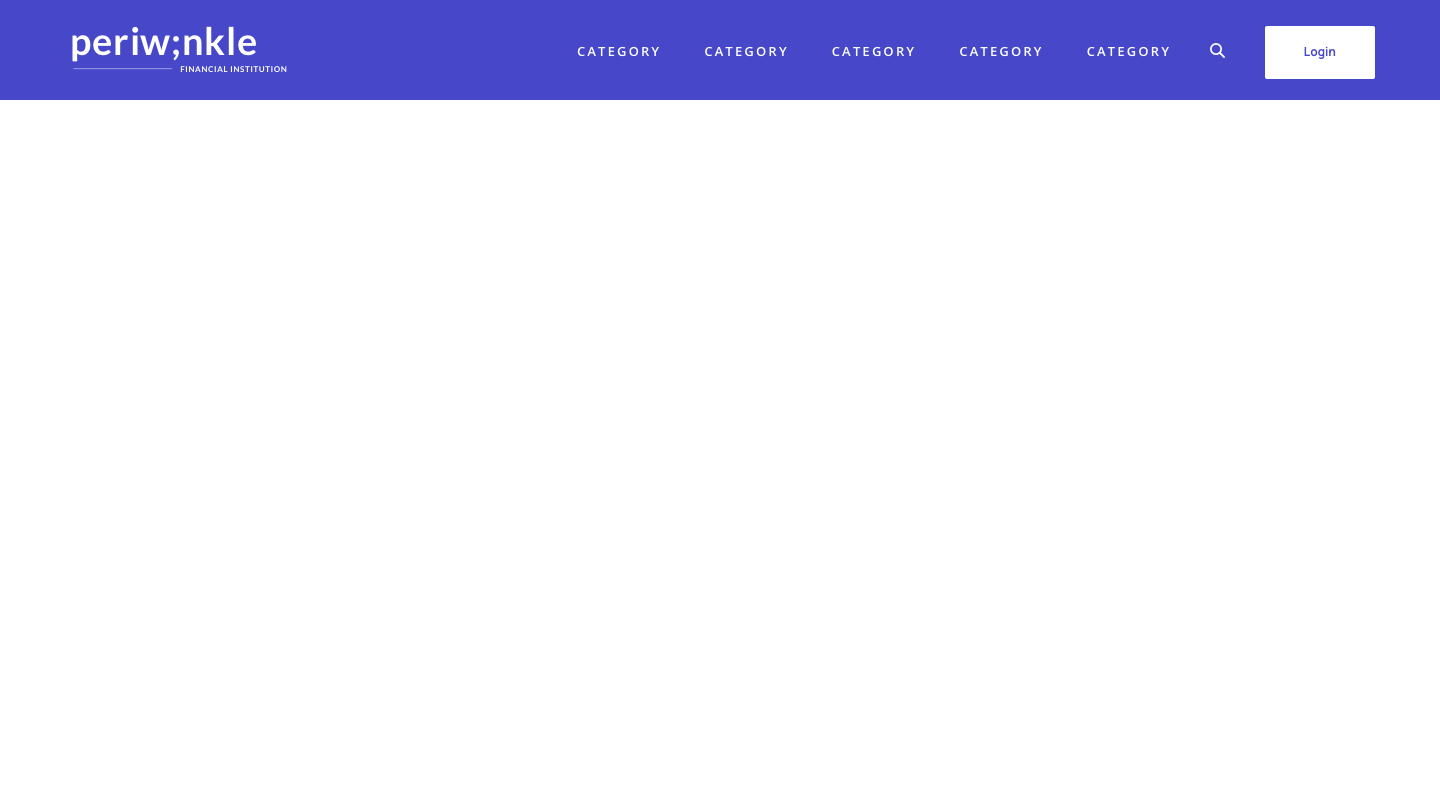A screenshot showcases the header section of a partially constructed website, likely created using a website builder or as a practice exercise for honing web development skills. The header features "Periwinkle" prominently as the title. On the left side, the text reads "Financial Institution," suggesting a theme related to banking or finance. The navigation menu includes repetitive placeholders labeled "Category," indicating that the final content isn't yet determined. Additional elements include a search icon and a blue "Login" button, providing minimal interactive features. The design employs a clean white background with blue text, emphasizing simplicity and ease of readability. Overall, the image portrays an early-stage, boilerplate template that requires further development to evolve into a fully functional website.